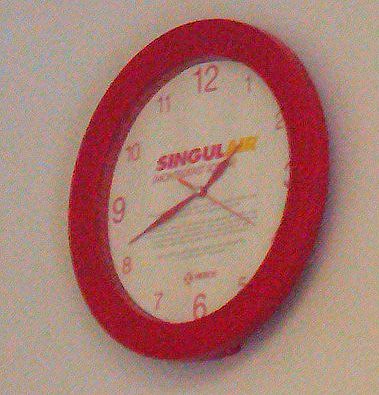This is an image of a distinctive red clock mounted on a beige wall. The image appears somewhat grainy, potentially a deliberate effect. The clock has a medium to dark red outer ring, with red numerals marking the hours. Notably, the numbers 12, 3, 6, and 9 are significantly larger than the other numbers. The clock's hands, including the second hand, are also red. 

Beneath the clock, the name of a prescription medicine is displayed. The word "SINGULAR" is split into two colors; the first part "S-I-N-G-U-L" is in red, while the remaining "AR" is in yellow. At the bottom of the clock's face, the brand name "MERCK" is prominently printed in red. Between the medicine name and the brand, there is additional text likely providing information about the drug. 

The clock's current time shows approximately 1:43.